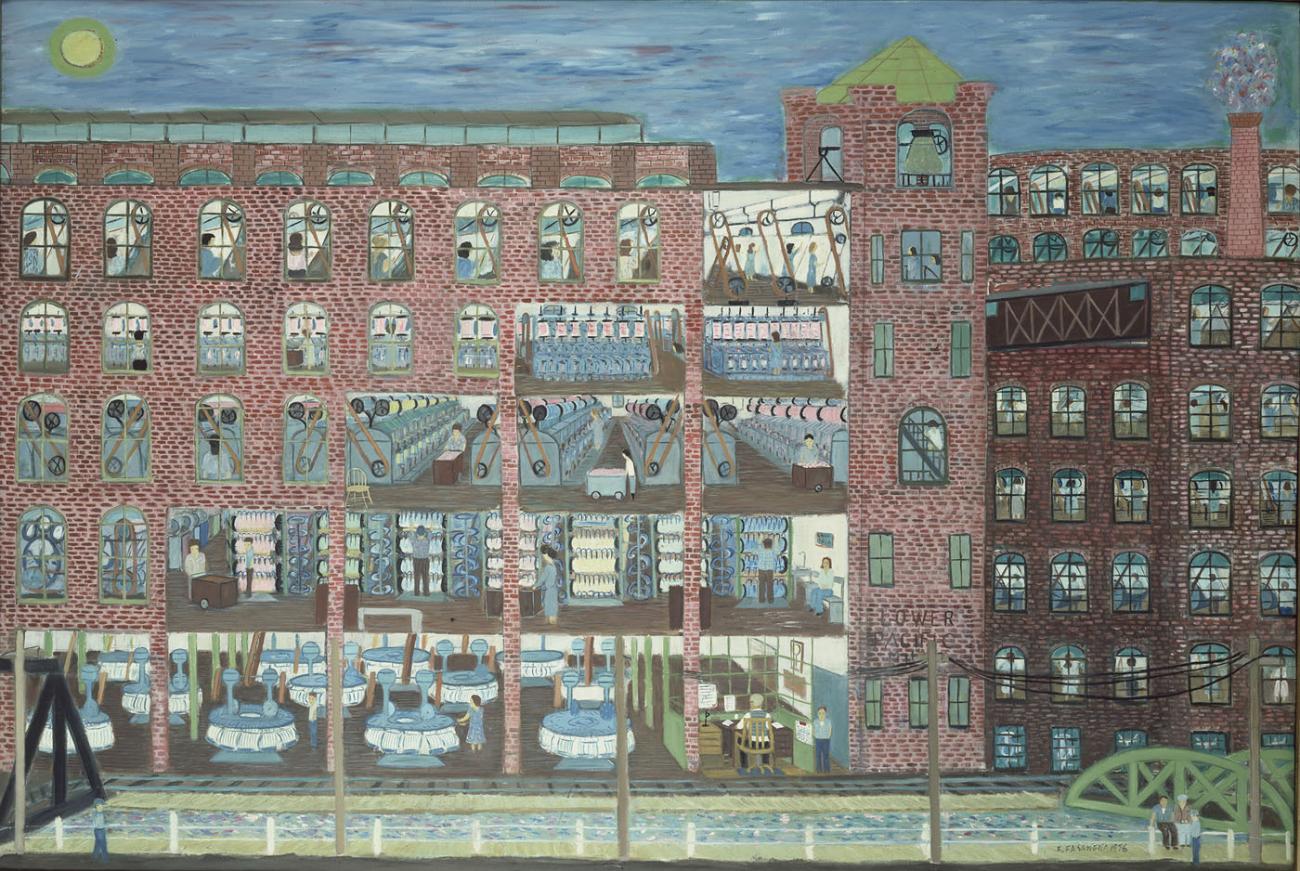This color painting by Ralph Fasanella, titled "Mill Worker, Night Shift, 1976," portrays a detailed, multi-story brick building from a landscape perspective. The building is composed of beige, rose, and dark brown hues, and the painting showcases a vibrant array of colors, including shades of blue, purple, yellow, green, red, tan, brown, and white. The scene is quasi-surrealistic, with quasi-representational elements.

The focal point of the painting is the large brick structure, which spans from top to bottom and features approximately six floors. Each floor depicts different activities inside: from the top, people are seen handling a big sheet, followed by floors populated with various machinery, laundry, bottles, and shells. At the very bottom, there is a bustling café with numerous tables. On the right side of the building, a man is sitting at a desk.

In addition to the building, the foreground includes a light green strip with a white picket fence running horizontally across the painting and a metallic green bridge positioned in the bottom right corner. A tower structure extends vertically from about two-thirds across the image, adding to the intricate detail. The sky is a vivid blue with a yellow sun situated in the top left corner, emphasizing the surrealistic essence of the scene. Together, these elements create a rich, detailed depiction of an urban setting, possibly reminiscent of a place like downtown New York or Chicago.